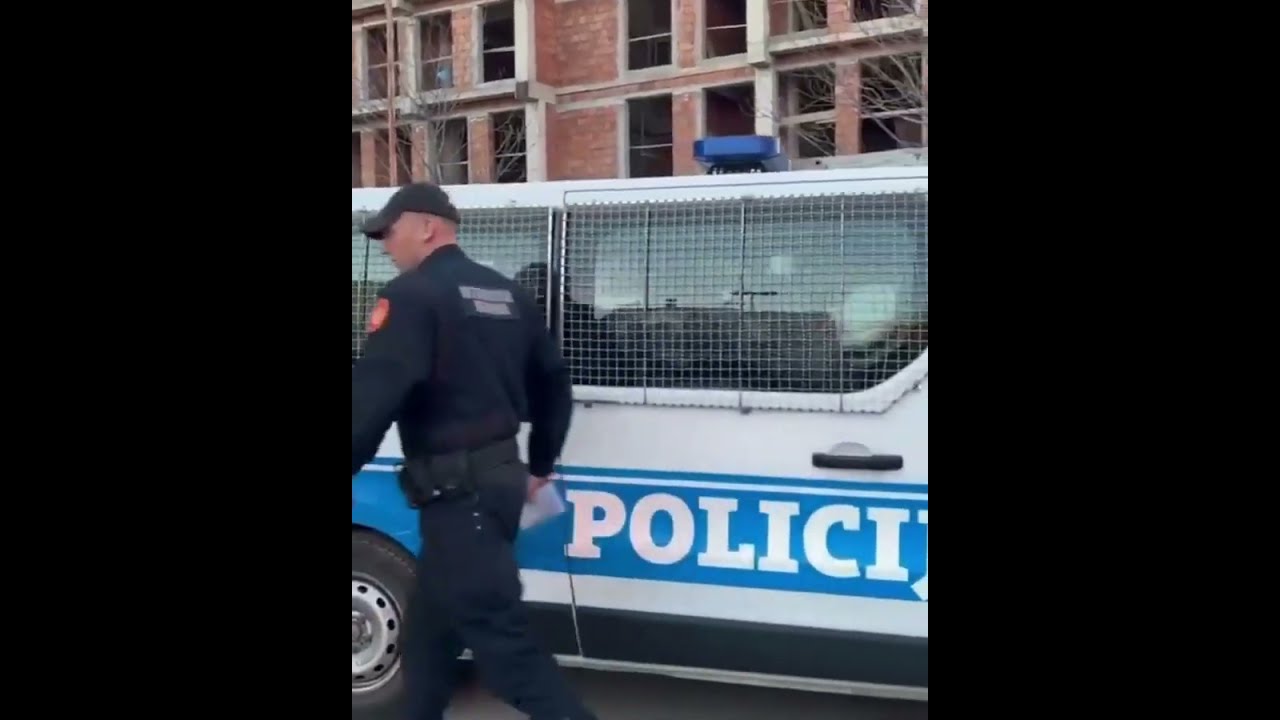The photograph features a white, multi-story, brick building with a slightly faded exterior. In front of it, there's a white police van, characterized by metal chicken wire bars covering its windows. The side of the van prominently displays a blue stripe with the word "POLICI" in bold white letters. To the left of the frame, partially out of focus, a bald, white police officer is walking toward the left. He's dressed in a dark blue uniform with matching pants, a black utility belt, and a navy baseball cap. Dominating the sides of the image are large black borders, almost as wide as the photograph itself, creating a stark contrast and framing the scene centrally.